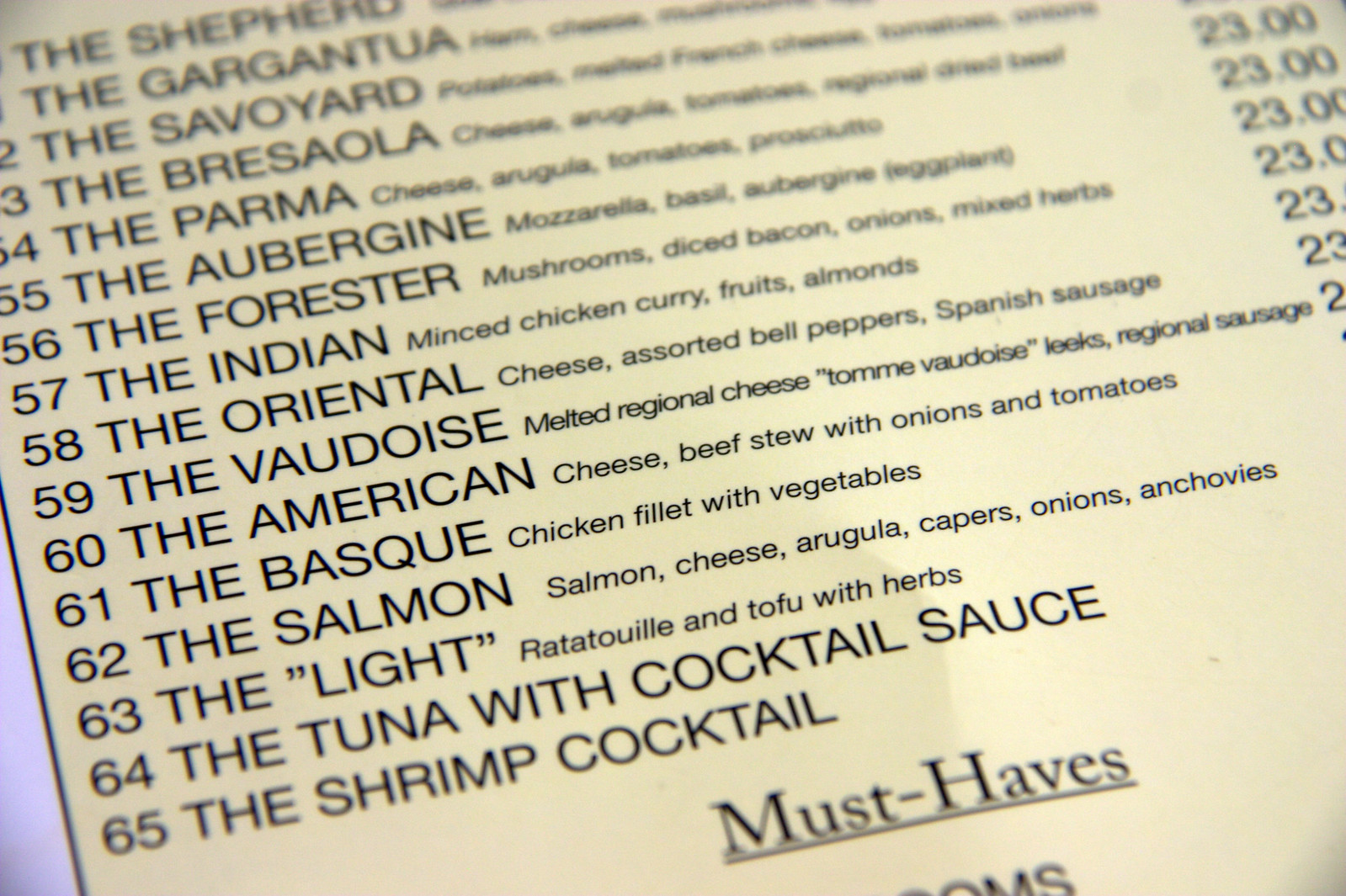The image depicts a close-up of a light yellow, potentially laminated menu displaying items with detailed descriptions. The visible section includes numbered entries from 55 to 65, showcasing a variety of dishes such as the Parma, the Aubergine, the Forester, the Indian, the Oriental, the Vaudois, the American, the Basque, the Salmon, the Light, the Tuna with Cocktail Sauce, and the Shrimp Cocktail. Each item is accompanied by its title and a brief explanation of its ingredients. All visible prices are set at $23. The menu displays a header titled "Must Haves" before the image cuts off. The off-white or light yellow hue of the paper and the slight shadow suggest overhead lighting when the photo was taken.